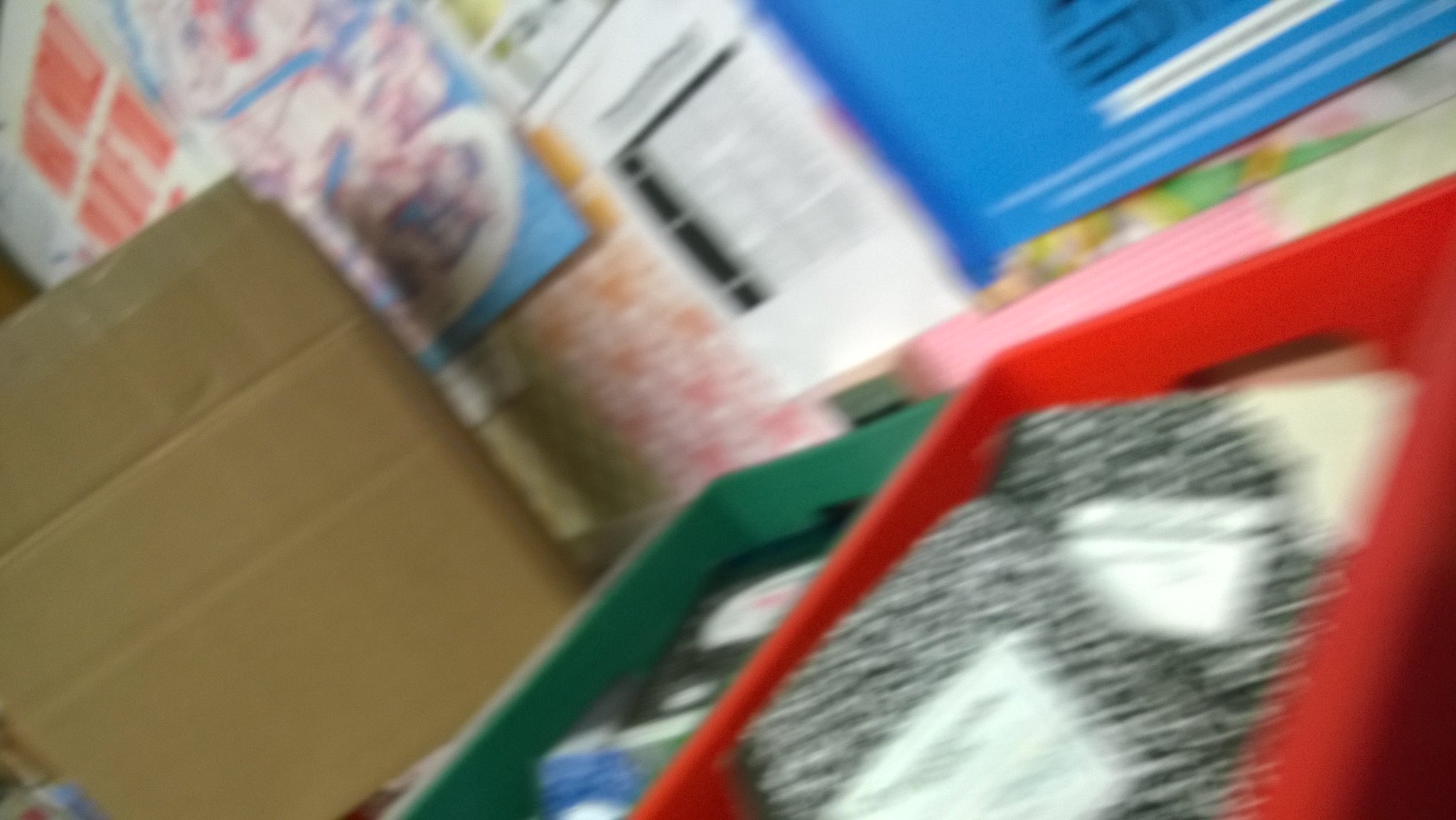In a slightly tilted and blurry image, a cluttered classroom scene unfolds. At the center, two milk crates - one red and one green - stand out. The red crate, positioned in the foreground, holds several black and white composition notebooks, some haphazardly thrown in. In contrast, the green crate is neatly packed, though its contents remain indistinguishable. To the left, a large cardboard box adds to the sense of either packing up for summer or unpacking supplies. The vibrant bulletin board behind is adorned with an array of colorful and less colorful posters, suggesting an educational environment rich with activity and information.